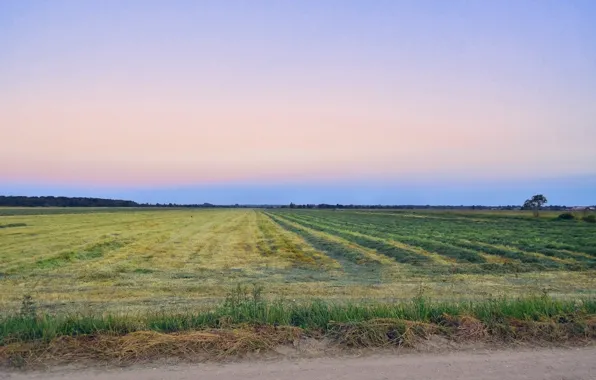This color photograph captures an expansive agricultural landscape under a stunning, multihued sky. The scene is split horizontally, with the sky taking up the upper half of the rectangular frame. The sky gradient transitions from a lighter blue at the top to hints of pink in the middle, turning into a darker, purplish hue near the horizon. The bottom half showcases a large field with distinct divisions: the left side is covered in yellowish, dry grass, while the right side features neat rows of short green crops or weeds. The foreground reveals a dirt road edged by a blend of green and dead brown weeds, some of which are flattened, suggesting recent disruption. A fence runs through this area, with clusters of tall grass surrounding it. In the distance on the horizon, a faint line of trees is visible, completing this picturesque rural vista.